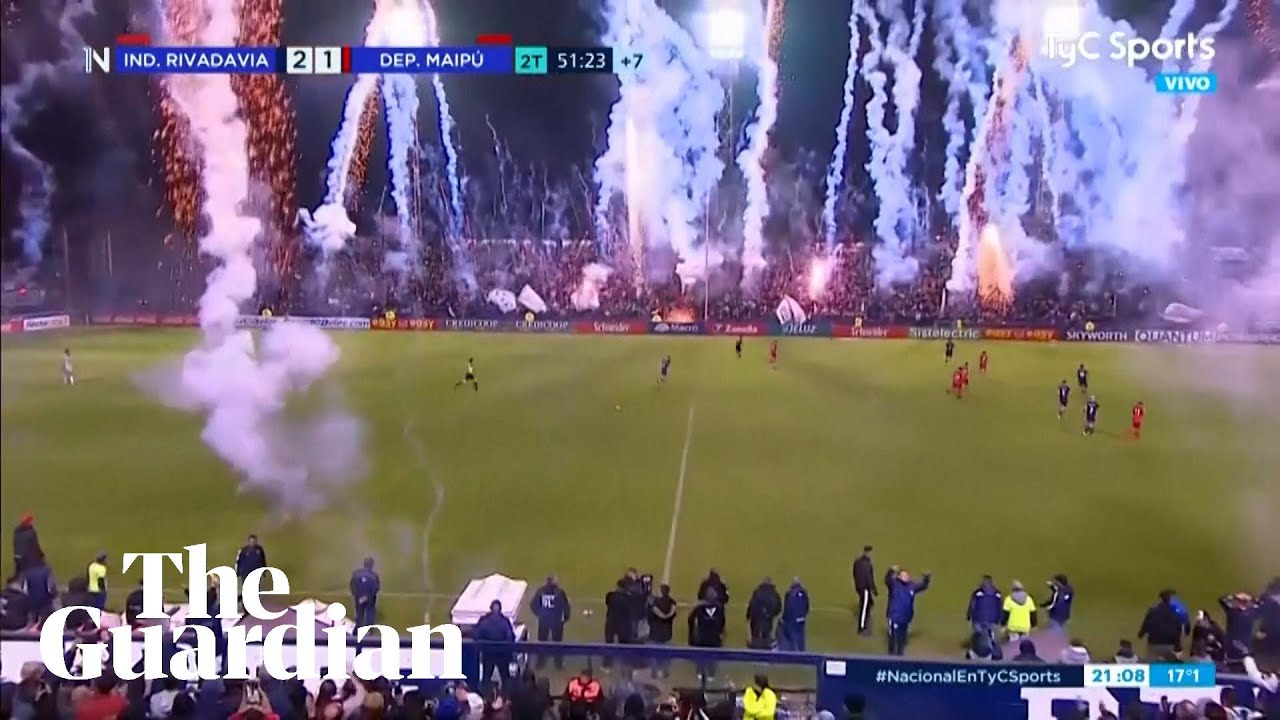This vibrant nighttime photograph captures the exhilarating atmosphere of a soccer match between Inderivadavia and Depmapu. The heavily contested game, currently at 51 minutes and 23 seconds into the second term, shows Inderivadavia leading 2-1, as indicated on the scoreboard in the top left corner. The top right corner of the image displays the "TYC Sports" logo with a blue "Viva" emblem. The match is being aired on "LYC Sports," as visible from the top right corner branding. Meanwhile, the Guardian newspaper's logo is prominently featured in the bottom left corner in white font.

At the heart of the image, fireworks burst spectacularly into the night sky, emanating from the audience areas. Plumes of smoke and glowing sparks trail vertically, dramatically illuminating the scene. The enraptured crowd fills the stands, cheering on the action unfolding on the field below. Players, distinguishable by their blue and red uniforms, are seen in dynamic motion, running towards the soccer ball. The sidelines are populated with team members and coaching staff, donning blue and black attire. This image is dominated by the explosion of fireworks, lending a festive energy to the thrilling match.